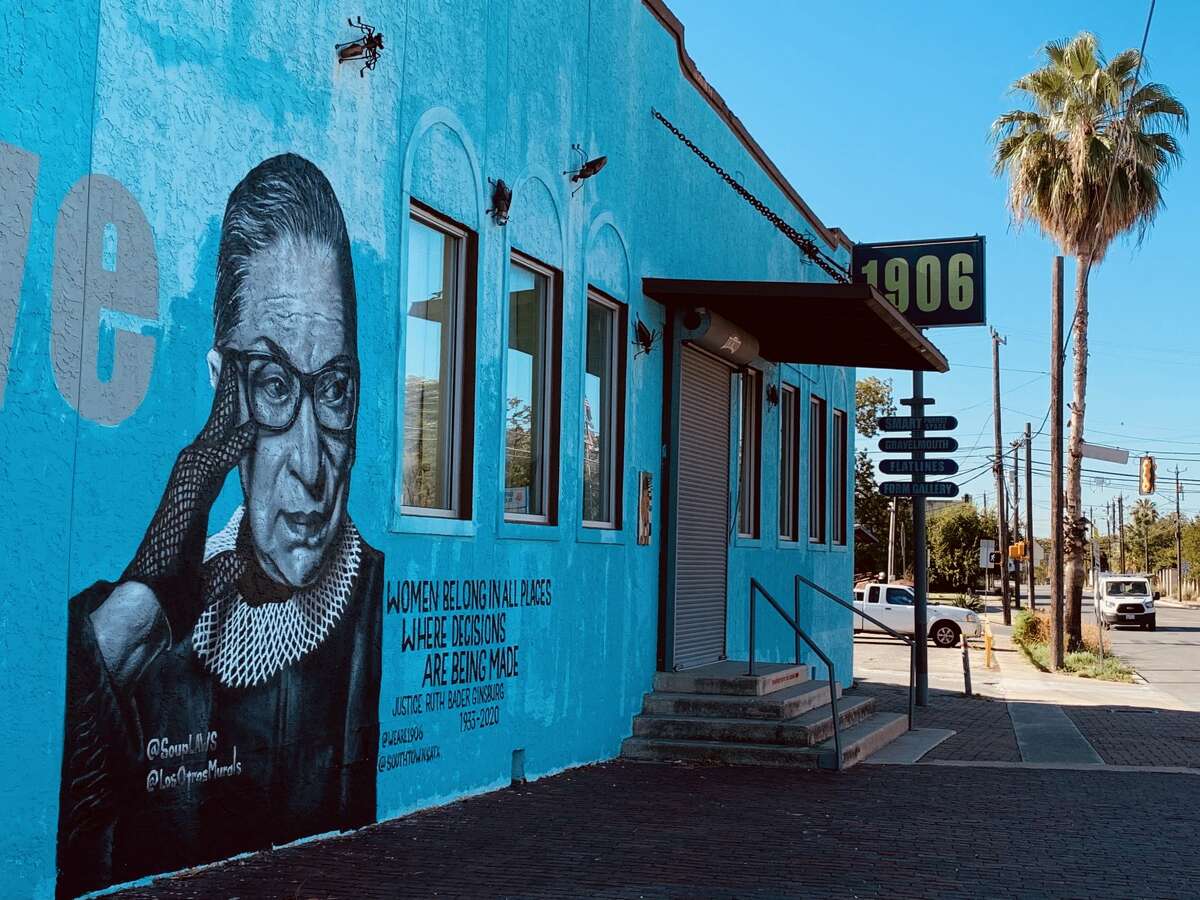Depicted is a vibrant outdoor scene on a sunny day featuring a one-story blue building with unique characteristics. Prominently, the left side of the building showcases a mural of Justice Ruth Bader Ginsburg, illustrating her with glasses, dark hair tied back, and dressed in a black judicial robe with lace gloves. Her hand is thoughtfully resting against her face. Accompanying this artwork is a significant quote in black text: "Women belong in all places where decisions are being made." Below the quote, her name and life span, "Justice Ruth Bader Ginsburg, 1933-2020," are inscribed. Above the building's entrance door, a sign reads "1906" in yellow letters. Adding to the building's distinctive appearance are three windows on each side of the door and four large plastic black bugs positioned above these windows. 

In the foreground, the scene includes a palm tree adjacent to a grassy sidewalk, adding a touch of greenery. A white truck is parked in a nearby lot, while a white van travels along the asphalt road in front of the building. The overall setting suggests an old, somewhat worn-out neighborhood, evidenced by the description of the area as "ratty" or "beat-up." Traffic lights are also visible among the background details, indicating a bustling yet nostalgic urban environment, all under a clear blue sky.